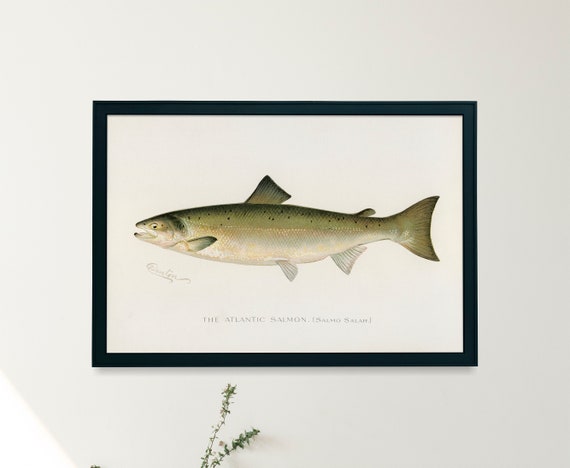This photograph showcases a detailed painting of an Atlantic Salmon (Salmo Salar) viewed from the side. The painting, encased in a sleek black frame, hangs against a light gray wall, which is consistently colored except for a small triangular patch of white light at the bottom left corner. The salmon's body is depicted with a greenish hue on the dorsal side, transitioning to light brown and hints of light orange on the ventral side. Every aspect of the fish, from its open mouth and eyes to its fins and tail, is portrayed with intricate detail. Below the fish, "The Atlantic Salmon" is written in black, followed by "Salmo Salar" in parentheses. Additionally, the artist's name is subtly mentioned on the left side, though it's not clearly legible. At the bottom of the painting, two narrow sprigs of vegetation with small, spiky green growths can be seen, adding a touch of natural life to the composition. The entire piece comes together to create a visually striking homage to the Atlantic Salmon.